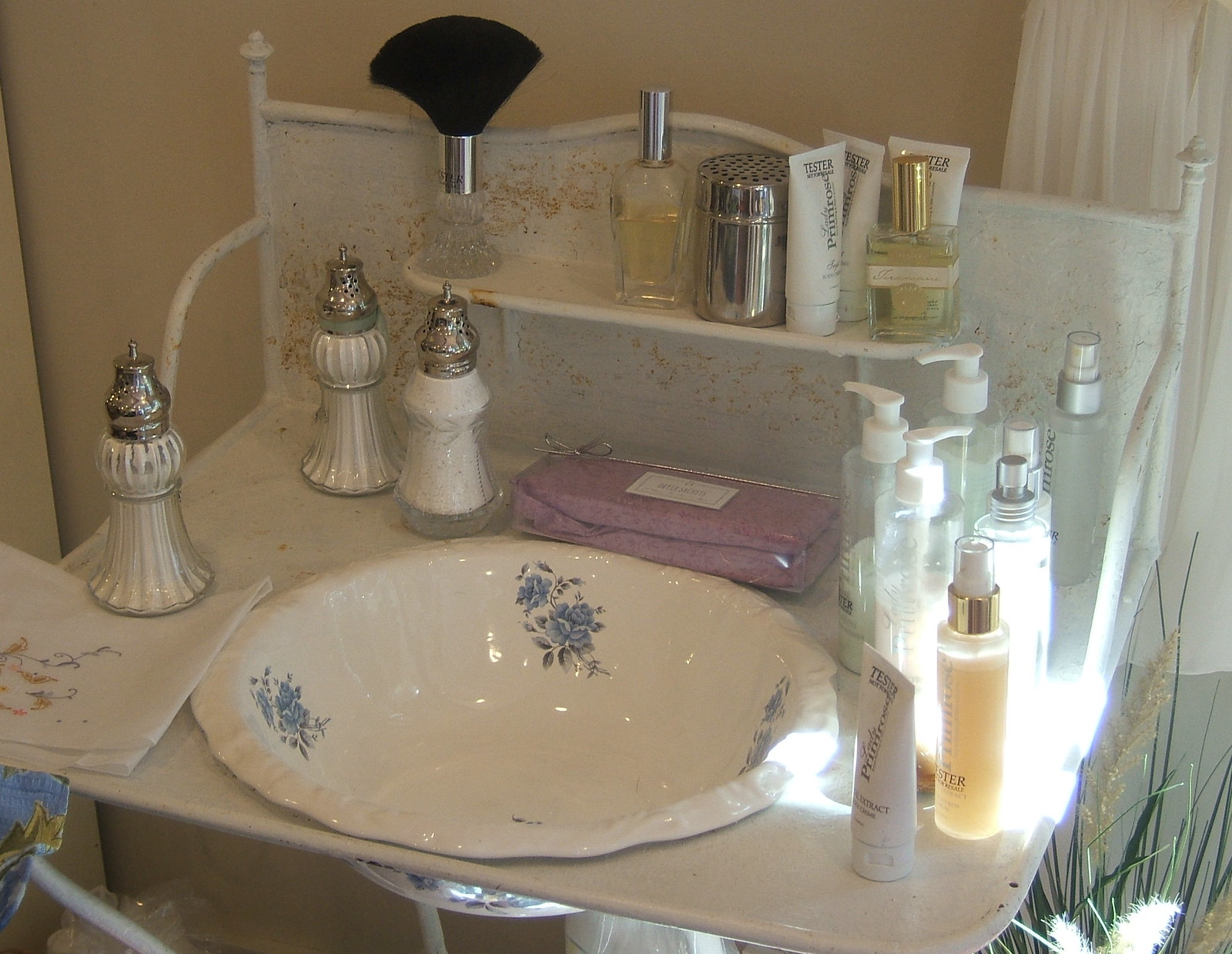The image is a color photograph showcasing a Victorian-style dressing table used as a bathroom basin. The basin itself, made of ceramic and inserted into a metallic surface, features a worn enamel finish with a blue flower motif around its inside edge. The photo is taken from a 45-degree angle slightly above, allowing a clear view of the basin's underside as it extends through the table surface, indicative of an old-fashioned design where water would be manually filled and emptied.

The table is cluttered with an array of beauty and bathroom products. On the left is a folded handkerchief, held down by what looks like a ribbed glass container, possibly a salt shaker, partially off-screen. There are two similar containers and one plain glass container, all holding some form of white powder that could be talcum powder or a beauty product. The centerpiece of the table is a collection of various bottles and pumps, including glass perfume bottles with silver and gold screw lids, modern squeezy tubes of moisturizer, and lotions. A small upturned makeup brush with a silver handle and black bristles rests on a vertical back shelf, adding to the vintage charm. Despite the lack of a mirror, the tabletop and shelf bear an organized chaos typical of a well-used vanity-turned-bathroom-basin from a bygone era.